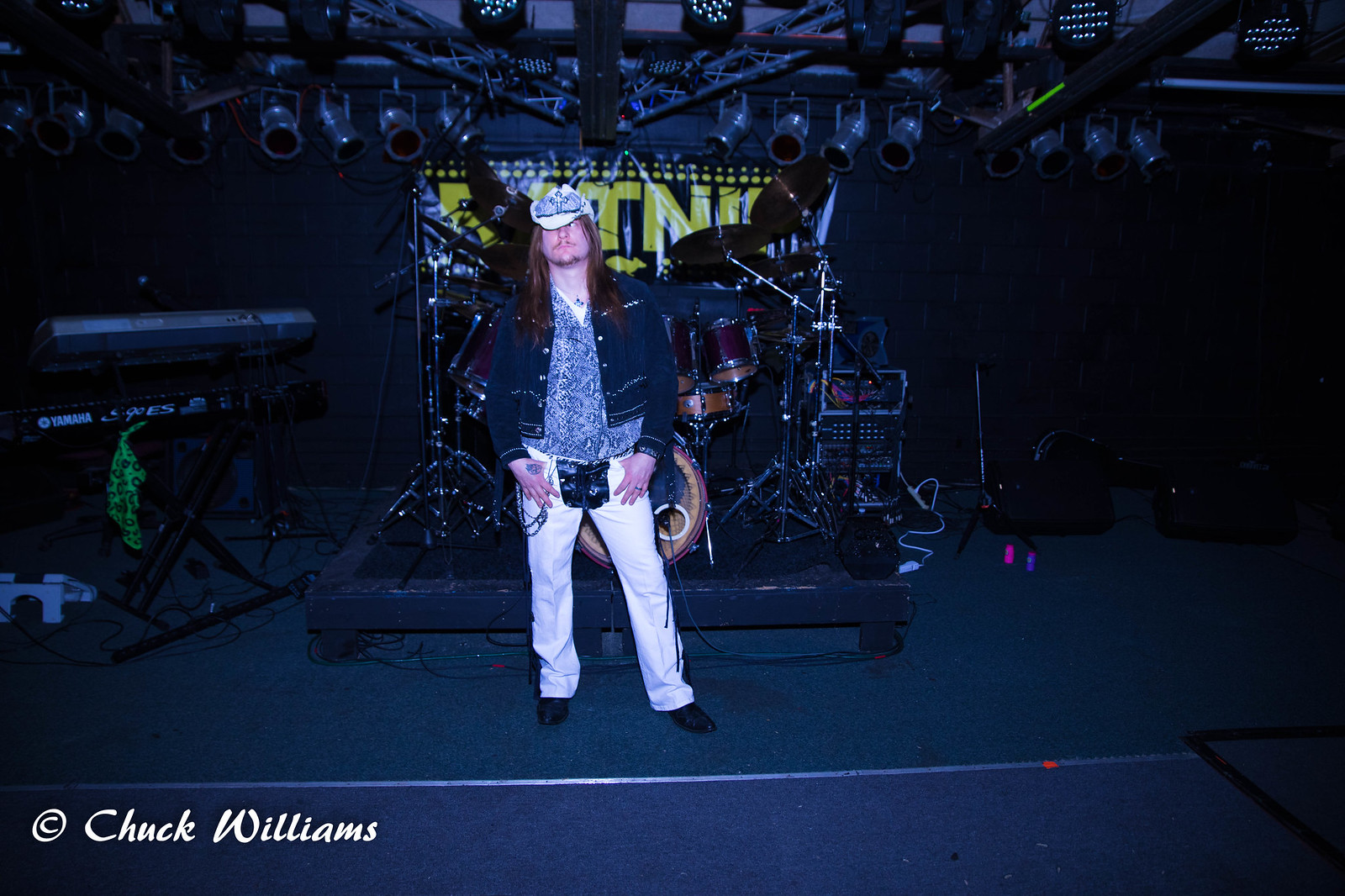In this indoor photograph, a man with long brown hair and a mustache, paired with a beard that extends under his chin, stands center stage. He is outfitted in a striking ensemble that includes black cowboy boots, white pants, and layers of blue clothing—a blue leather jacket over a blue vest, which itself is layered over a white undershirt. Atop his head rests a white cowboy hat adorned with a cross. Behind him, a drum set complete with chimes takes up the central stage space, flanked by keyboards or synthesizers adorned with a green or black bandana on the left and electronic music equipment on the right. Above the scene, numerous spotlights are poised but currently off, hinting at a stage set for performance. The backdrop consists of a dark brick wall with a partially obscured yellow poster displaying indiscernible text in the background. In the bottom left corner, the photograph is marked with a white copyright notice reading “copyright Chuck Williams.”